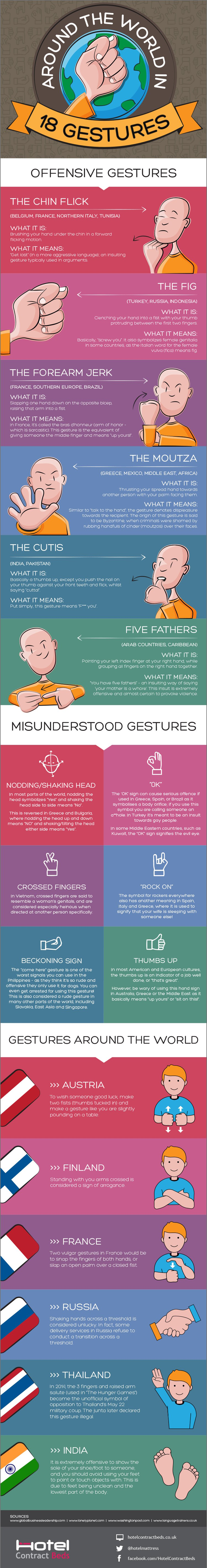The infographic is a tall, narrow, and visually engaging image titled "Around the World in 18 Gestures" set against a gray background. At the top, there's a circular logo in white featuring an illustration of the globe with a hand making a fist and thumb gesture, accompanied by a yellow banner displaying the title. Beneath the title, the infographic is divided into several categorized sections. The first section, labeled "Offensive Gestures" on a white banner with black text, features cartoon illustrations of various offensive hand gestures, each named and depicted by a cartoon character. Following this, a section titled "Misunderstood Gestures" is presented. The final segment, "Gestures Around the World," showcases various gestures alongside flags from different countries, including Belgium, France, Northern Italy, Austria, Finland, Russia, Thailand, and India. Each gesture is depicted in vibrant, colorful illustrations, though due to the image's small size, the details of the text are challenging to read. The infographic encompasses a comprehensive guide to culturally diverse hand gestures, though its intricate details are hard to discern at a glance.